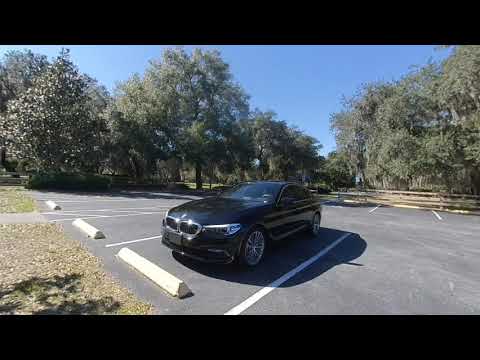This detailed photograph captures a black BMW, likely a newer model, parked in a vacant parking lot on a bright, sunny day. The BMW, characterized by its signature grill and chrome trim around the front, is neatly positioned within a white-lined parking space, flanked by cement barriers designed as speed bumps. The parking lot, with its dark gray pavement and tidy layout, stretches out with freshly mowed grassy areas tinged with light yellow and brown hues on either side. Surrounding the lot are numerous trees, their green foliage silhouetted against a vivid blue sky. In the background, a gray sidewalk leads off into the distance, emphasizing the tranquil, organized setting that suggests this could be the parking area of a park. The shadows cast by the trees and the car indicate that the sun is shining from the left side of the image, enhancing the serene daytime atmosphere. The photograph is presented with a narrow black header and footer, adding a subtle frame to the scene.